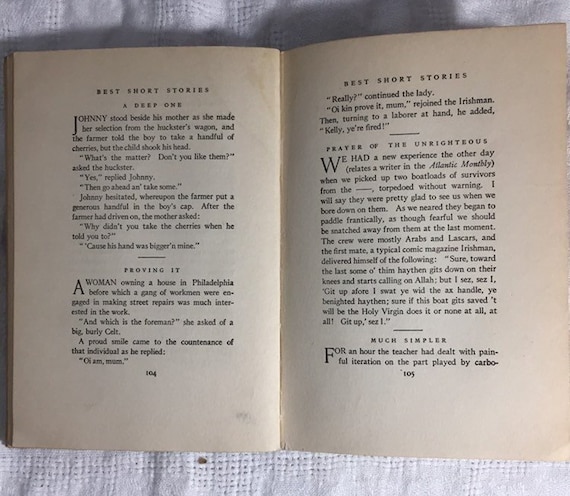The square image shows an open book, specifically pages 104 and 105, revealing the titles and excerpts of short stories. The book appears to be older, as indicated by its discolored, light tan pages, which bear the stains and yellowing typical of aging paper. The text on both pages is in black and is justified in alignment. Page 104 features the titles "Best Short Stories" with subsequent stories "A Deep One" and "Proving It," each followed by paragraphs. Page 105 continues with "Best Short Stories," followed by the titles "Prayer of the Unrighteous," consisting of a long paragraph, and then "Much Simpler" with a brief text. The book is placed on a white, porous cloth, possibly a napkin or blanket, which shows tiny dots cut out at the top and bottom, adding texture to the background. The top part of the cloth casts a shadow from the book, suggesting the presence of daylight on the right side of the image.